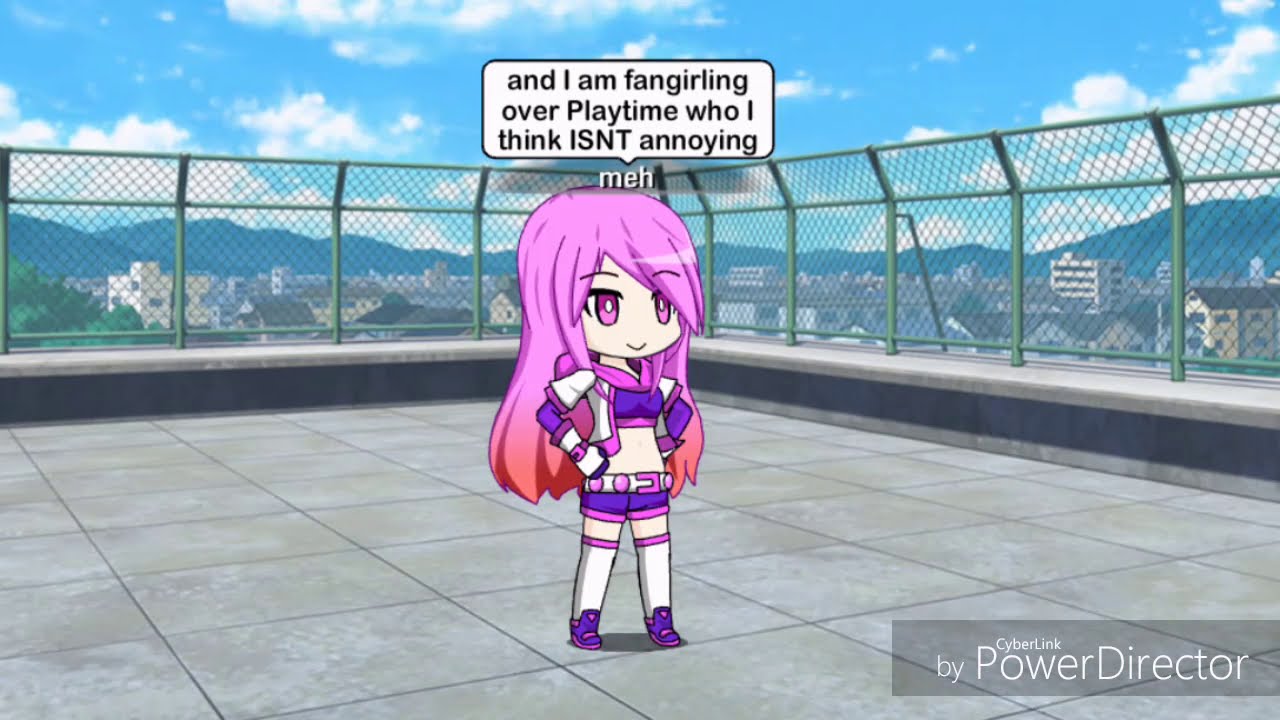This image features a chibi-style anime character standing on a rooftop, enclosed by a curved green chain-link fence for safety. The rooftop has tiled concrete flooring and a concrete barrier. The character has long pink hair that is frosted with red tips and she is adorned in a trendy outfit consisting of a purple tube top, a white and pink shirt, a matching white and pink belt, and purple shorts. She completes her look with white and pink high socks that go above her knees, long white gloves, and purple running shoes. She sports purple eyes and a pink-lined vest with a hood. Above her head, a white speech bubble with black text reads, "and I am fangirling over Playtime, who I think isn't annoying." In the background, you can see a cityscape with numerous buildings, a mountain range, and a blue sky dotted with white clouds. On the bottom right corner of the image, the text "Cyberlink by PowerDirector" is displayed in a rectangle.